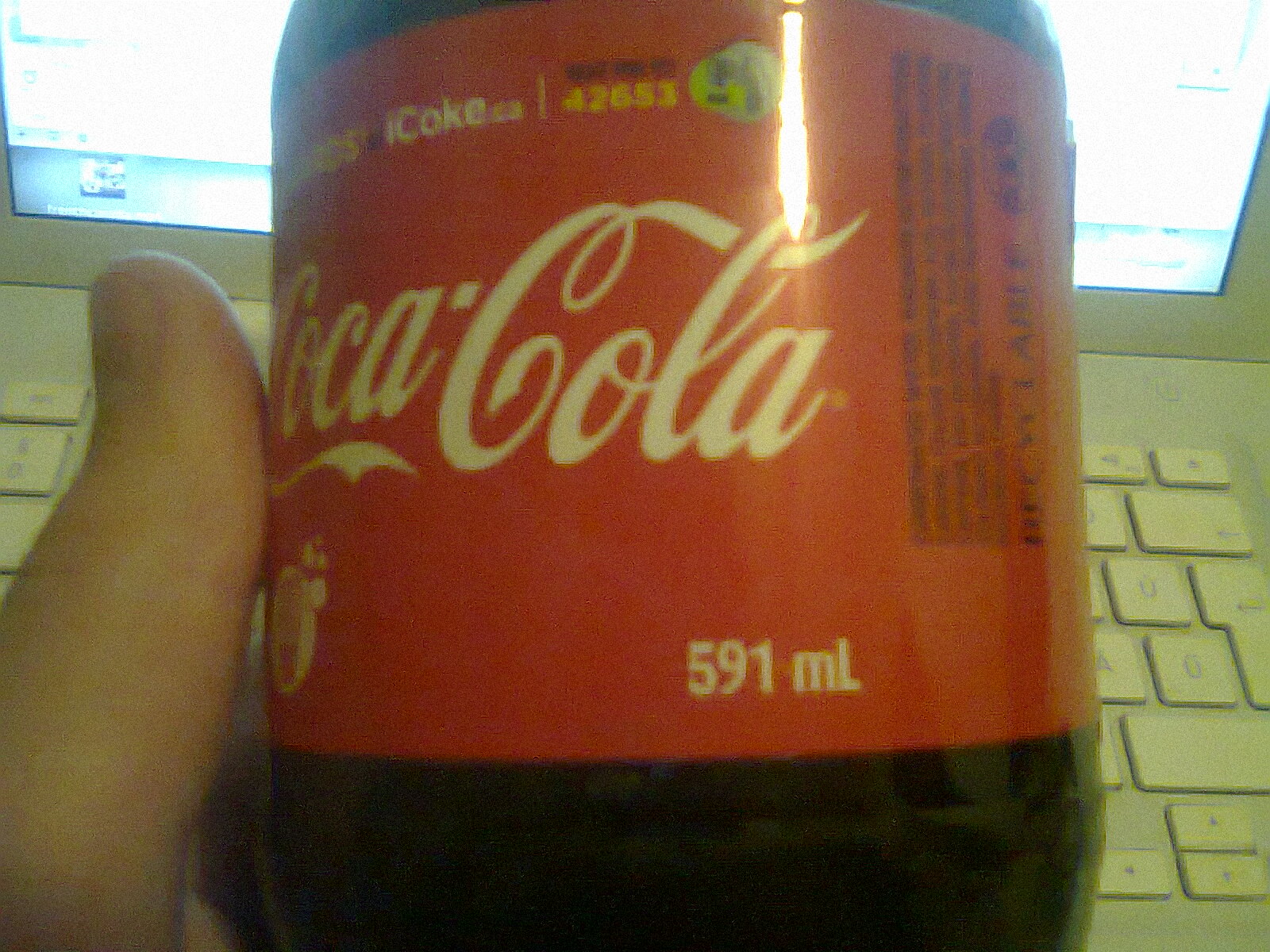This close-up image captures the side of a Canadian Coca-Cola bottle, clearly identifying it as a plastic container. The iconic Coca-Cola logo is prominently displayed on the left side of the bottle. A person's thumb is visible, holding the bottle upright for the photo. The lower right corner of the label indicates the volume as 591 milliliters. At the top of the label, there's additional text mentioning iCoke.ca, reinforcing that this is a Canadian product. The bottle also has a lot number, 42653. In the background, a white keyboard is visible, suggesting the presence of an open laptop, evidenced by the screen and the keyboard below it.